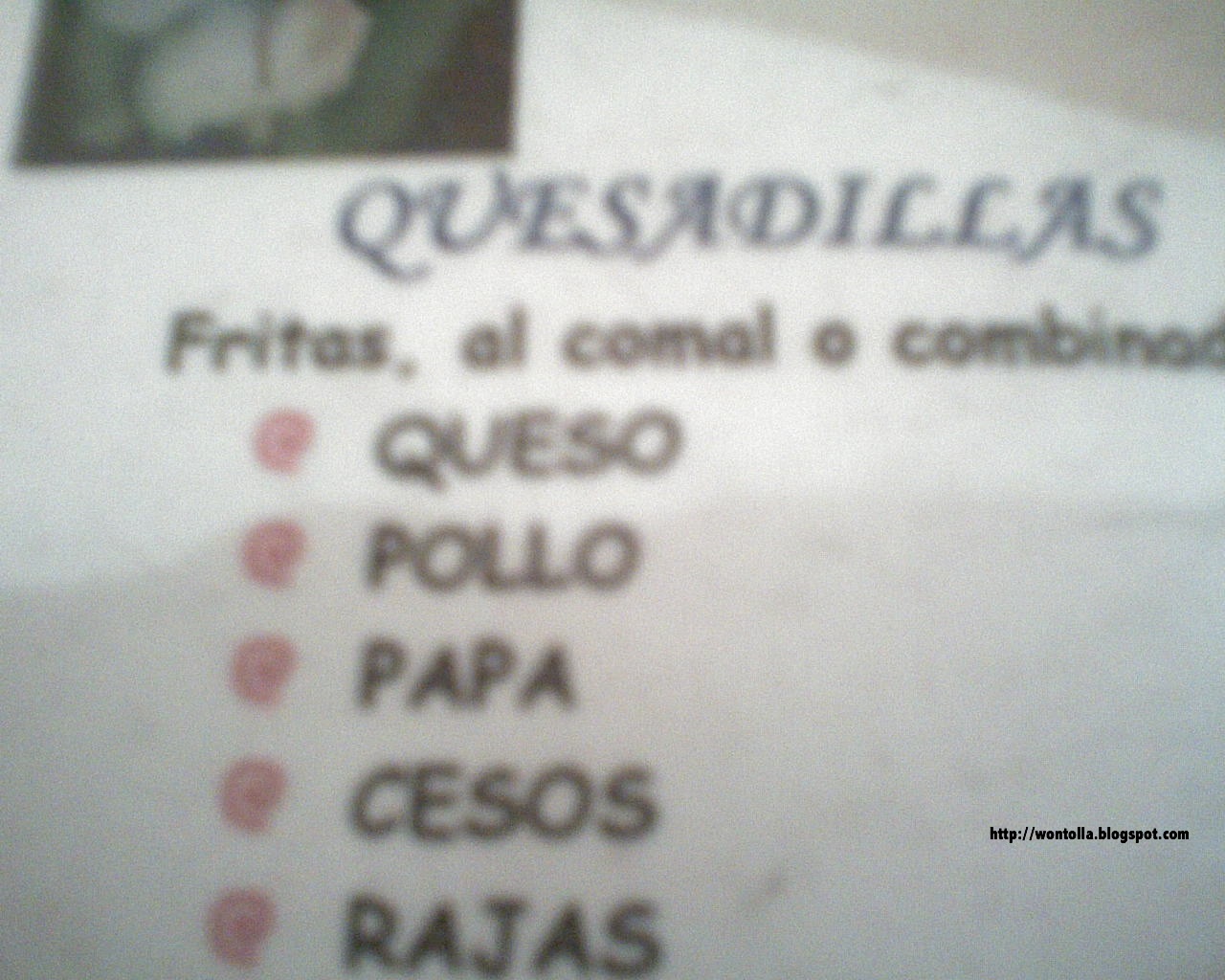A slightly out-of-focus photograph showcases a white menu. In the upper left-hand corner of the menu, there's a square photo with a green background and indistinguishable white elements. Below the photograph, in a navy blue uppercase font, the word "QUESADILLAS" is prominently displayed. Underneath this heading, in black font, it reads "Frida's Cama El Combinado," although the word "Combinado" is truncated at the edge of the photograph. Below this, five items are listed, each preceded by a small red bullet point: "QUESO," "POLLO," "PAPA," "QUESOS," and "RAJAS," all in uppercase letters. In the lower right corner of the photograph, there's a small text that reads "http://blackspot.com."